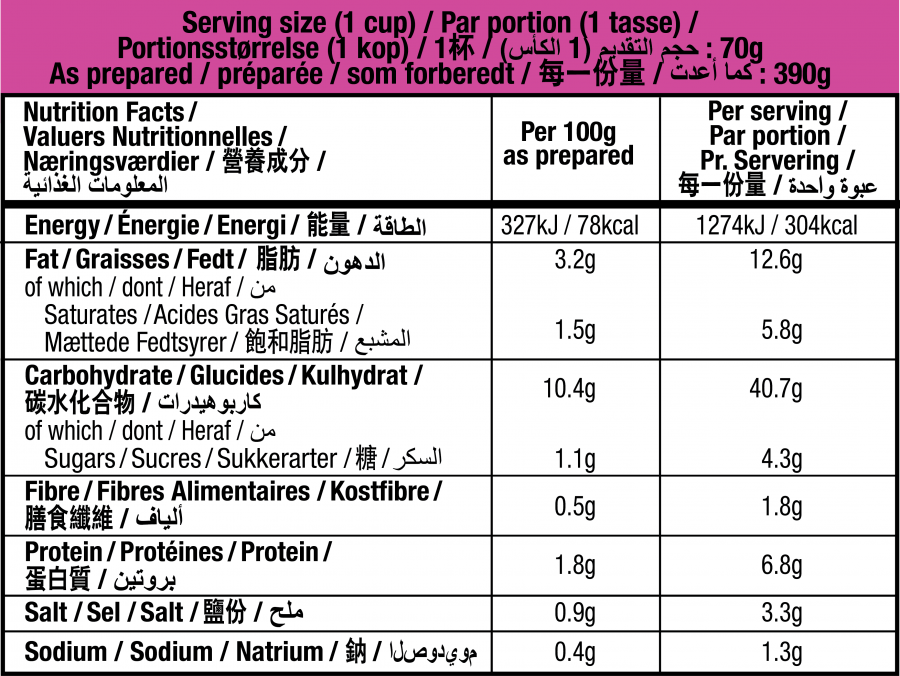Detailed Caption: 

This image showcases a detailed nutrition label, prominently featuring a purple header with clear, black text. The label provides essential nutritional information for a serving size of 1 cup. Notably, the information is presented in multiple languages, enhancing accessibility for a diverse audience. Key details include measurements in two formats: per 100 grams as prepared and per serving. For instance, the energy values are listed as 327 kJ per 100 grams and 1274 kJ per portion. Fat content is specified as 3.2 grams per 100 grams and 12.6 grams per serving, with saturated fat being 1.5 grams and 5.8 grams respectively. The carbohydrate content is noted as 10.4 grams per 100 grams, with fiber at 0.5 grams. Additionally, protein amounts to 1.8 grams, salt is 0.9 grams, and sodium is 0.4 grams per 100 grams of the prepared product. This label offers a comprehensive overview of the product's nutritional profile, allowing consumers to make informed choices.